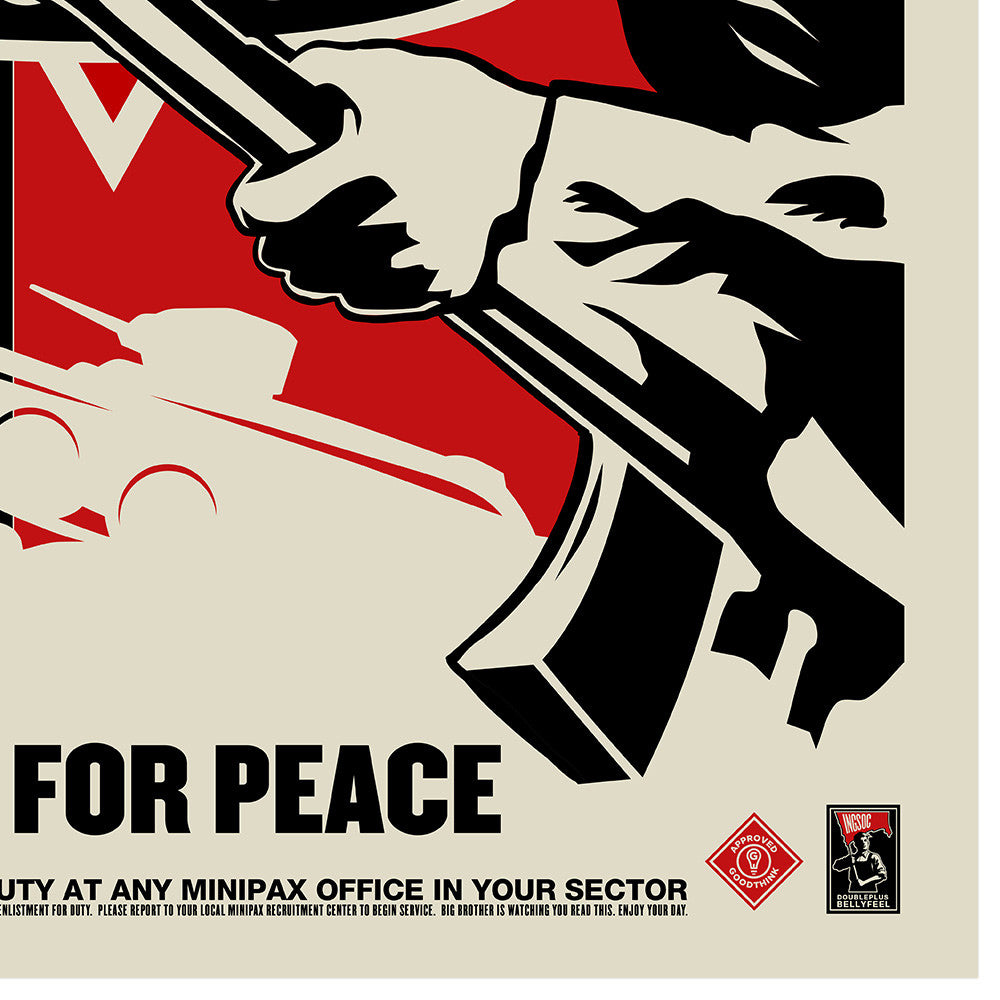The lower portion of the poster is predominantly white, red, and black. On the right-hand side, bold black text reads "FOR PEACE." Below it, larger fragmented text shows "DUTY at any MINIPACS office in your sector," followed by smaller, less legible writing that includes "please report to your local MINIPACS recruitment center to begin service." Distinctively, a red diamond-shaped emblem stating "APPROVED GOODTHINK" with a circle and a light bulb featuring the letter "G" appears nearby. To its right is a square logo of INGSOC, depicting a gentleman holding a flag with white writing on a red background. The poster's design includes a graphic of a hand gripping a military rifle, partially visible in the foreground, and a white silhouette of a tank against the red backdrop. At the very bottom, the text reads "DOUBLE PLUS BELLY FEEL," emphasizing the propagandistic and ideological nature of the artwork.